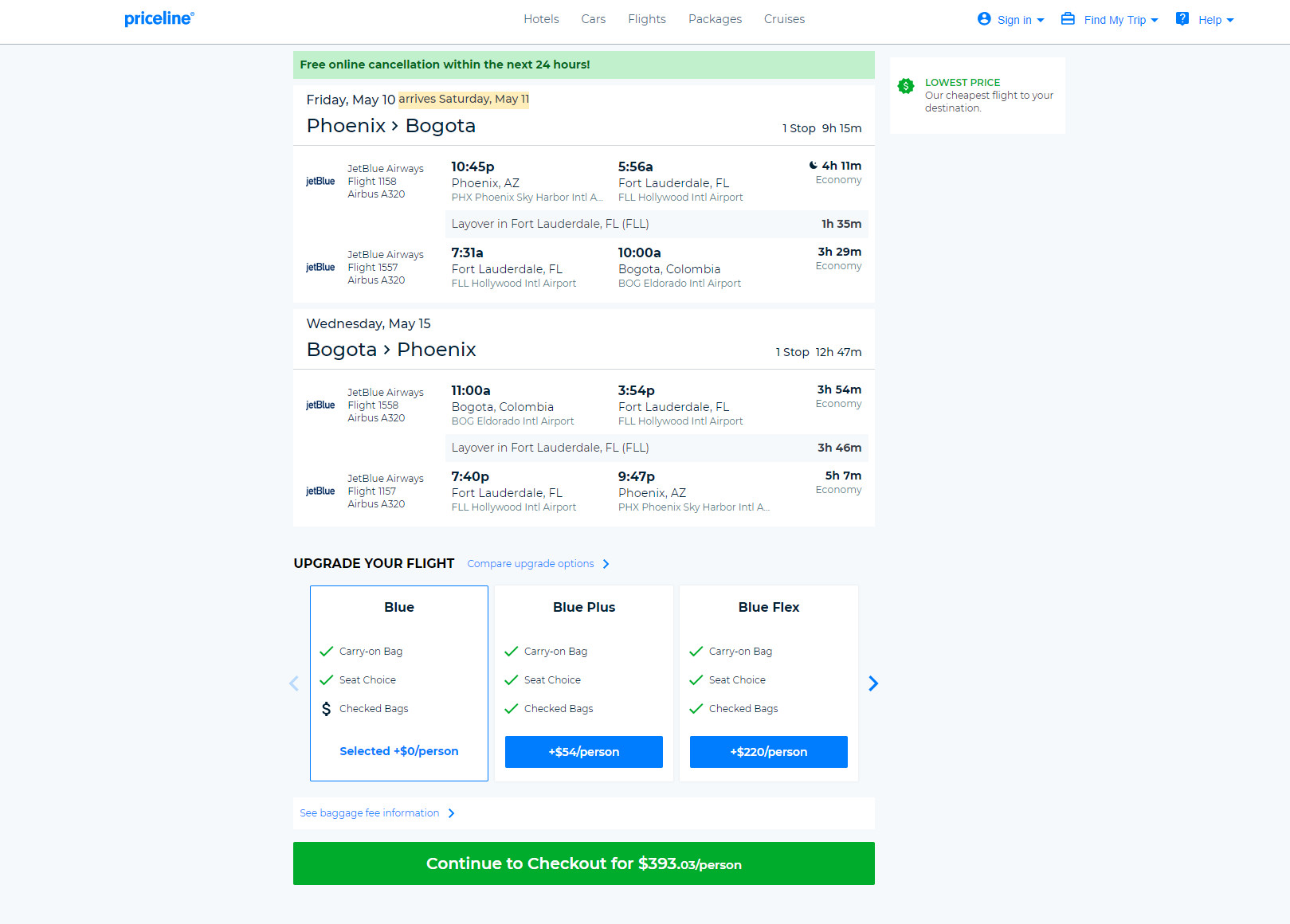The screenshot from the Priceline website features a sleek layout with a white background at the top. On the left, the blue Priceline logo, and at the center, black tabs for various booking categories: hotels, cars, flights, packages, and cruises. On the right, blue menus for "Sign In," "Find My Trip," and "Help."

Beneath this, a light blue background showcases a white central area with pivotal information. A green banner at the top announces in black text: "Free online cancellation within the next 24 hours." Below this, on the white background, detailed flight itinerary information is displayed.

For Friday, May 10th with an arrival on Saturday, May 11th, the highlighted dates mark the journey from Phoenix to Bogotá. There are two listed flights: 
1. **JetBlue Flight 1158**: Departing Phoenix at 10:45 PM and arriving in Fort Lauderdale at 5:56 AM.
2. **JetBlue Airways Flight 1557**: Departing Fort Lauderdale at 7:31 AM and arriving in Bogotá, Colombia at 10:00 AM.

For the return journey on Wednesday, May 15th from Bogotá to Phoenix:
- **JetBlue Flight 1558**: Departing Bogotá at 11:00 AM and arriving in Fort Lauderdale at 3:54 PM, followed by:
- **JetBlue Flight 1157**: Departing Fort Lauderdale at 7:40 PM and arriving in Phoenix at 9:47 PM.

Below the flight details, there are options to upgrade your flight. At the bottom of the screen, a button reads "Continue to checkout" with a cost of $393 per person.